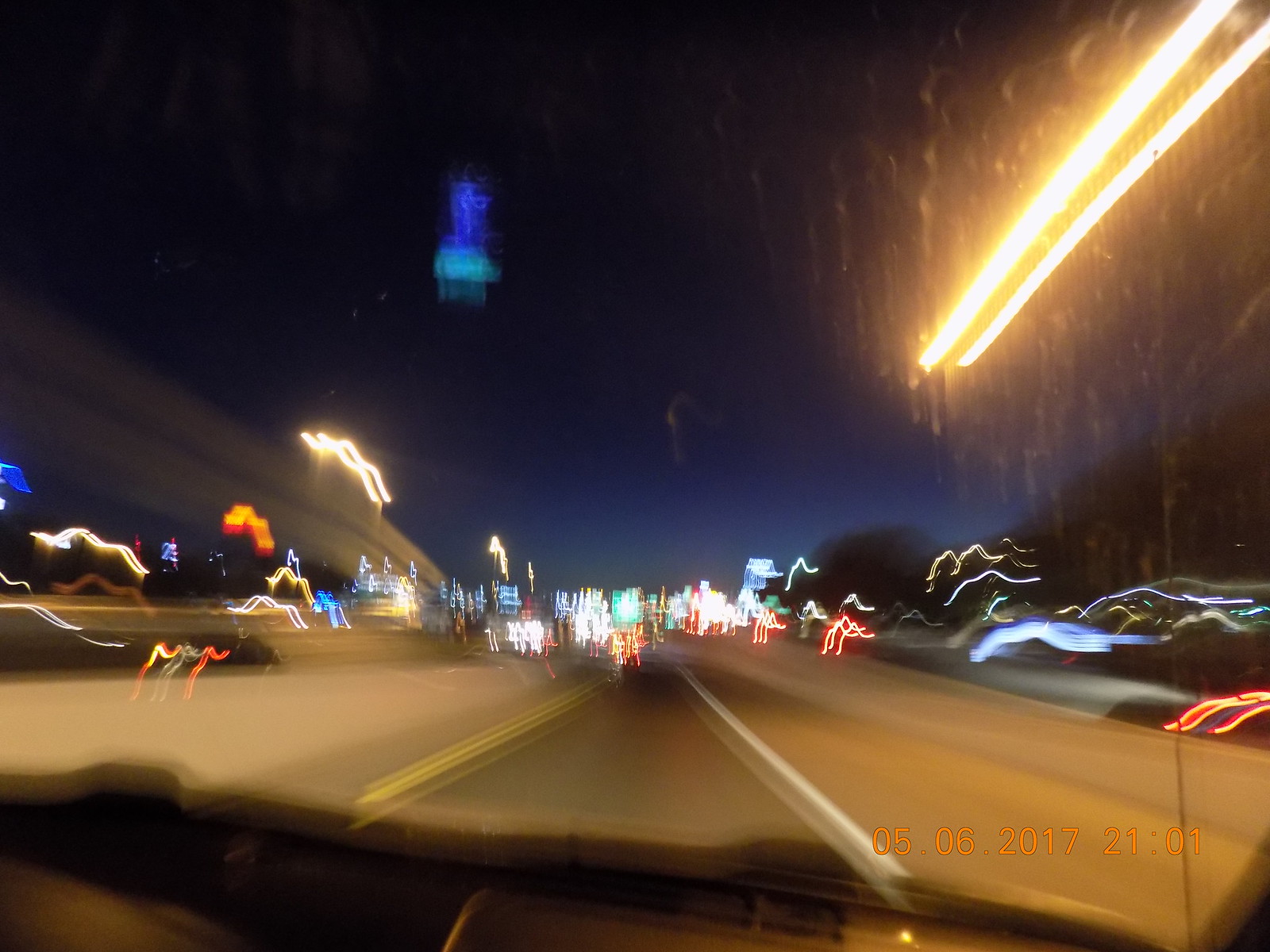A car is captured speeding down a road at night, seen from the perspective of its windshield. The scene has a surreal, almost AI-generated quality to it, with vibrant bolts of color resembling lightning striking both sides and the center of the road. These bolts, in a spectrum of neon colors, contribute to a psychedelic atmosphere. The night sky above is dark, and towards the top right corner of the image, a long, fluorescent light casts a pale yellow glow, reminiscent of lighting found in a garage. The light stretches from the top right corner into the background, adding an additional layer of depth and intrigue to the scene.